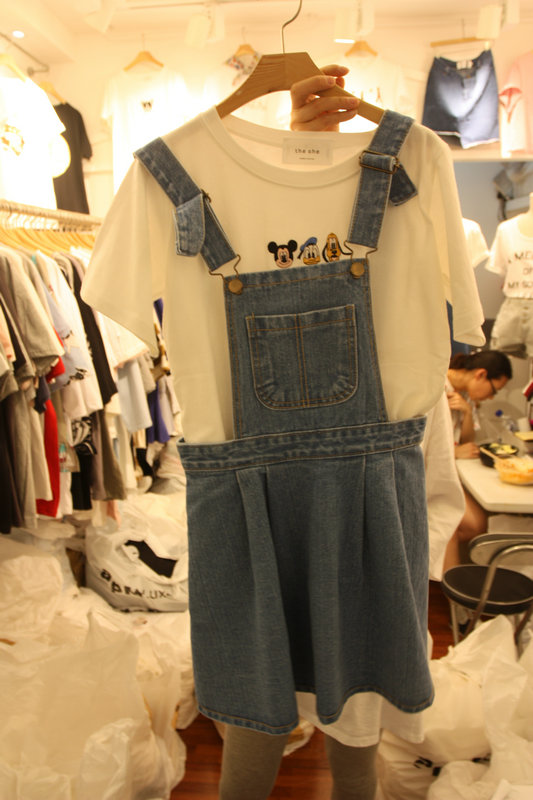The photograph, likely taken in a store's backroom based on the cluttered and informal setting, shows a hand holding up a white shirt adorned with Mickey Mouse, Goofy, and Pluto, layered beneath a blue denim skirt overall. The person holding the outfit is mostly obscured, with only their hand and feet visible. The backdrop reveals racks of colorful clothes on tan wooden hangers and white plastic bags scattered on the darker burgundy brown floor, possibly filled with additional clothing items. White walls and a white ceiling frame the space, with various garments, including a visible blue jean skirt, hanging high. On the right side, a woman with black glasses and dark hair, possibly of Asian descent, sits at a white desk, seemingly engrossed in a task, hinting at this being a multi-functional, storage, or workspace area rather than a typical retail shopping section.